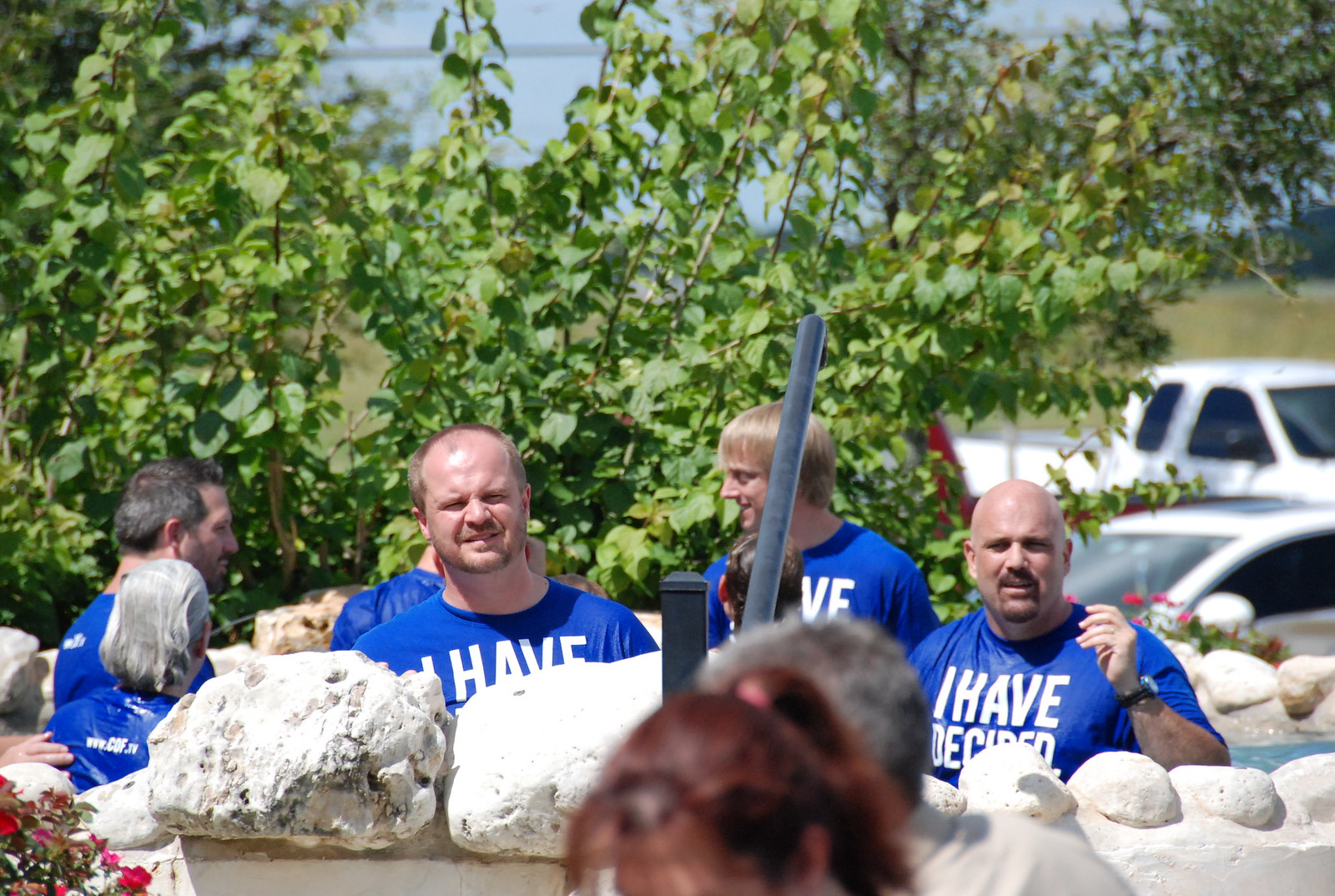The horizontal rectangular photograph captures an outdoor scene with multiple individuals all wearing matching blue t-shirts. Prominently displayed text on the shirts reads "I have decided," though the full message is partially obscured by a white and concrete stone wall in the foreground. Among the group, three men stand front and center; the one in the middle has hair, while the other two are bald, one sporting a mustache. Behind them, at least one woman with long gray hair can be seen next to a man with short hair and a beard. The background reveals lush greenery with large green leaves, a road with a white car and a white truck, and a noticeable brunette-haired woman in the foreground with a pink hair accessory. The overall color palette of the photograph consists of blue, green, and white, creating a vivid, coherent scene.